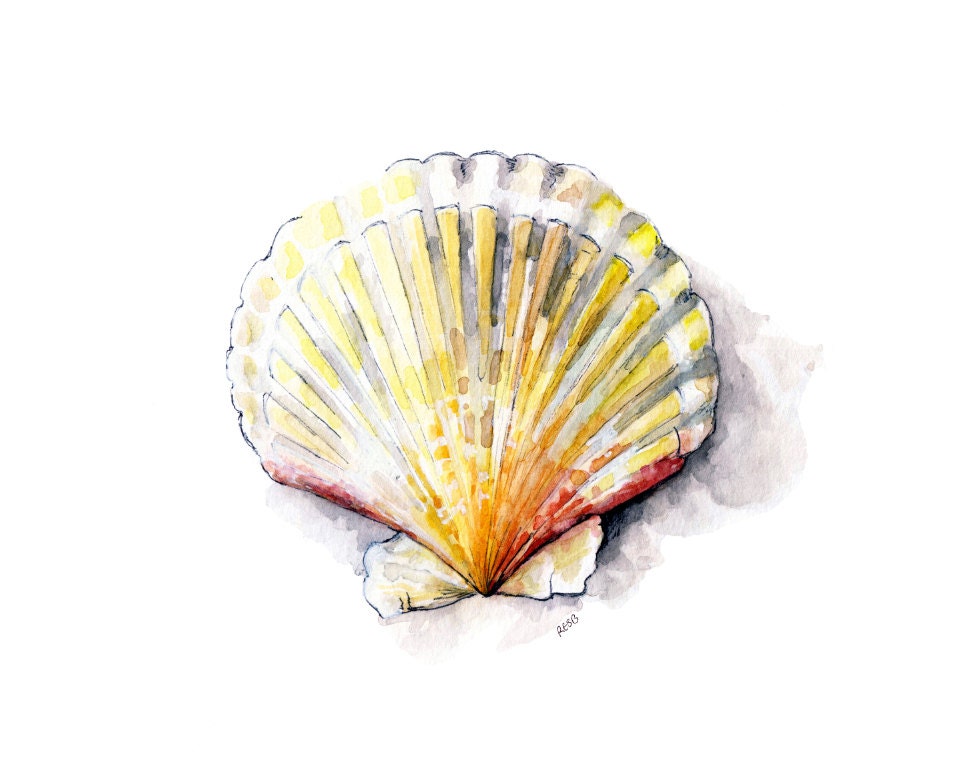This image depicts a watercolor drawing of a seashell, reminiscent of the fan-shaped scallop commonly associated with the Shell gas station logo. The shell is predominantly white, adorned with light to dark yellow lines that converge at the tip, with sporadic tinges of red, gray, and brown giving it a nuanced appearance. The colors slightly blend together with a subtle pen outline, enhancing its delicate detailing. At the bottom, there is an additional shape that resembles a bow tie, illustrated in similar hues of white and yellow. The shell is presented from an overhead perspective, creating a focused and intentional composition centered solely around the shell. The background features varying shades of gray, perhaps suggesting shadows, adding depth to the image. The artist has signed the piece "RESB" in the bottom right corner, affirming its creation. Although some may find the tie-dye-like color pattern reminiscent of kitschy designs, the artwork maintains a careful balance of colors and detail that highlights the shell's intricate beauty.